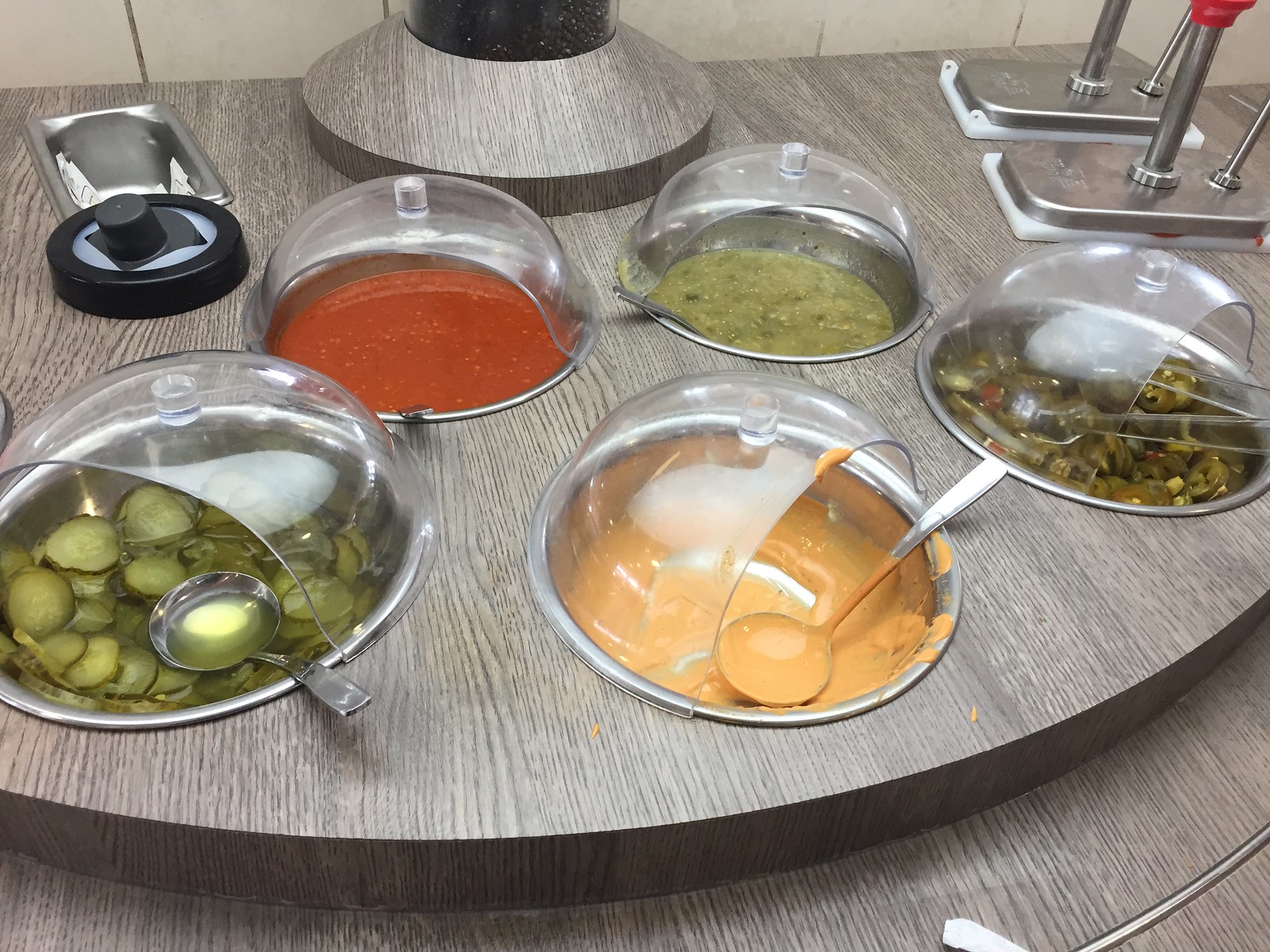The image depicts a buffet-style condiment station, situated on a wood grain finish laminate counter. The station features five stainless steel bowls, each partially covered with plastic lids that open on the side facing the bottom. Each bowl contains different food items and is equipped with a metal spoon for serving. The leftmost bowl holds pickles with a large silver spoon. Next to it is a bowl containing Thousand Island dressing, followed by one with green beans. In the back row, the far left bowl appears to contain either salsa or tomato soup, while the bowl next to it likely contains guacamole, each with its own serving spoon. In the upper right corner, there are two silver pump dispensers, likely for ketchup and mustard.